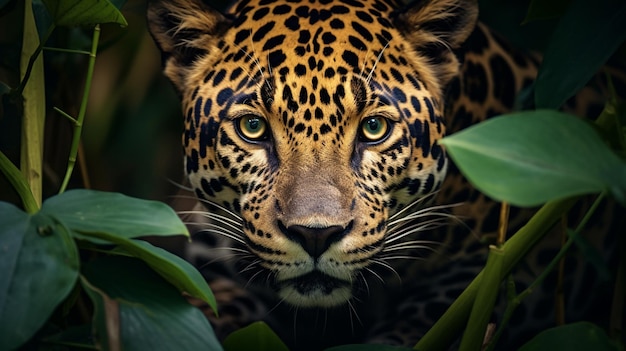This is a stylized digital illustration, likely AI-generated, depicting a close-up of a jaguar's face peering through dense jungle foliage at night. The jaguar's intense gaze locks with the viewer's, its golden eyes wide open and framed by short, triangular ears just visible at the top of the image. Its coat is an orangeish-yellow with dark brown spots and a darker snout. White whiskers sprout prominently from either side of its muzzle. The jaguar is partially obscured by green, waxy leaves and plant stems, adding to the sense of depth and enclosure in the scene. The background is almost entirely black, emphasizing the jaguar's striking features and the vivid colors of the foliage surrounding it.